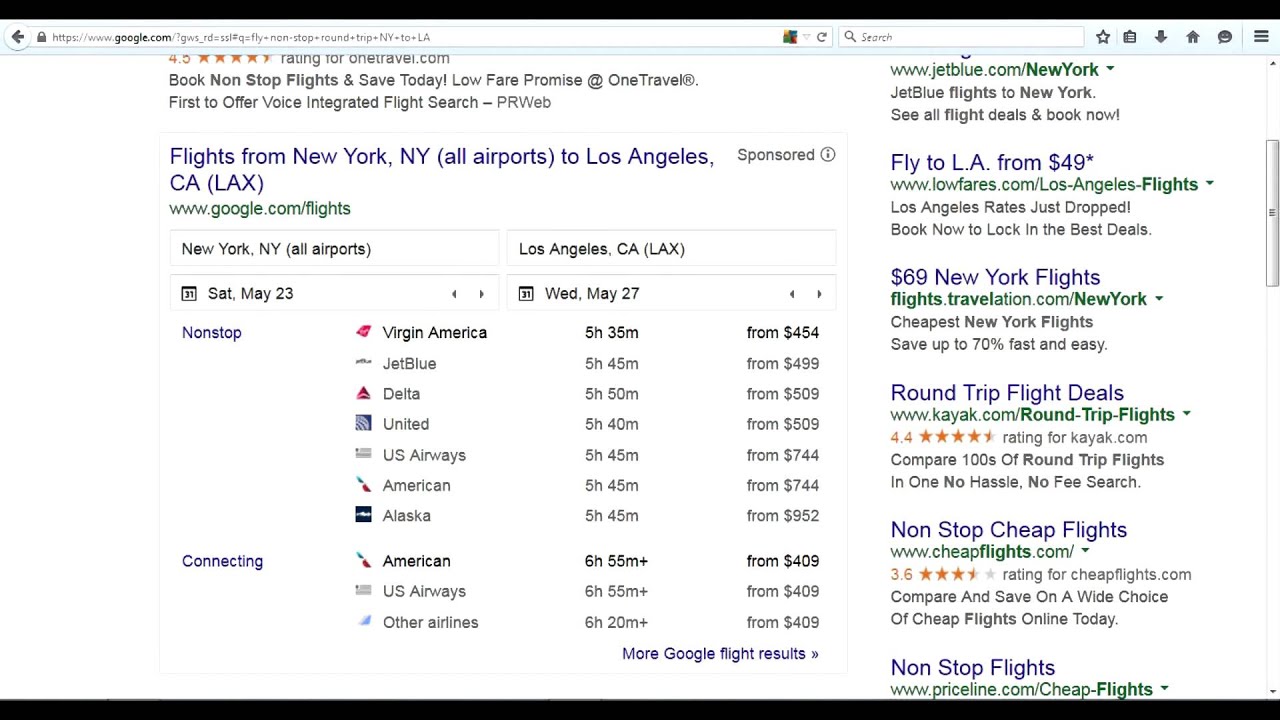This image captures a Google search results page, displaying the search query for flights from New York to Los Angeles. The screen is divided into two distinct sections: the left-hand column and the right-hand column. On the left side, the actual Google search results are shown, offering a variety of flight options. These include both connecting and nonstop flights, along with details such as flight dates, prices, airline names, and flight durations. Each option is presented in a clickable format, enabling users to make informed decisions easily.

The right-hand column, in contrast, is entirely dedicated to advertisements related to flight bookings. Several travel booking websites are promoted here, including Travelation, Kayak, CheapFlights.com, and Priceline.com. Each advertisement highlights different prices for round-trip flights, aimed at encouraging users to explore these external websites for potential deals. This dual layout efficiently presents both organic search results and sponsored content, providing a comprehensive overview for anyone researching flights between these two major cities.